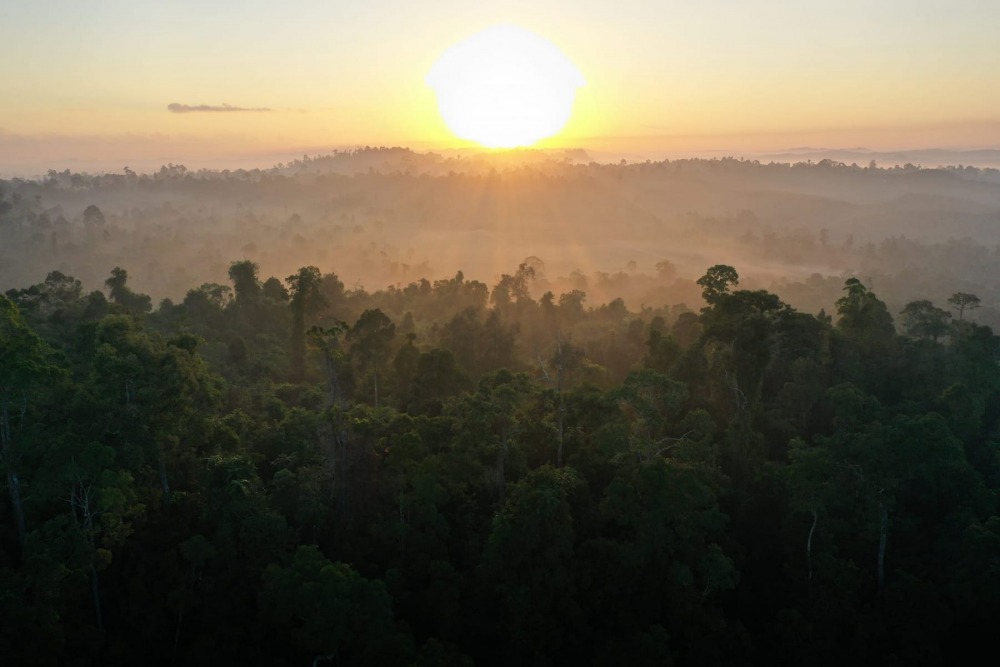This image captures a breathtaking sunrise over a dense, fog-kissed Amazonian jungle. The sun, positioned centrally at the top, radiates a bright white and yellow light, transitioning into warm hues of orange and pale reds as it illuminates the clear blue sky. A hillside descends into a lush valley filled with densely packed, tall trees of forest green, shrouded in a light fog. In the foreground, the great forest prominently stands, its dark greens contrasting with the vivid colors of dawn. A large body of water glistens beneath the sunrise, reflecting the serene beauty of the scene. The perspective suggests that the photo was taken from an elevated vantage point, likely a drone or helicopter, offering a sweeping vista of the Amazonian wilderness awakening to the new day.